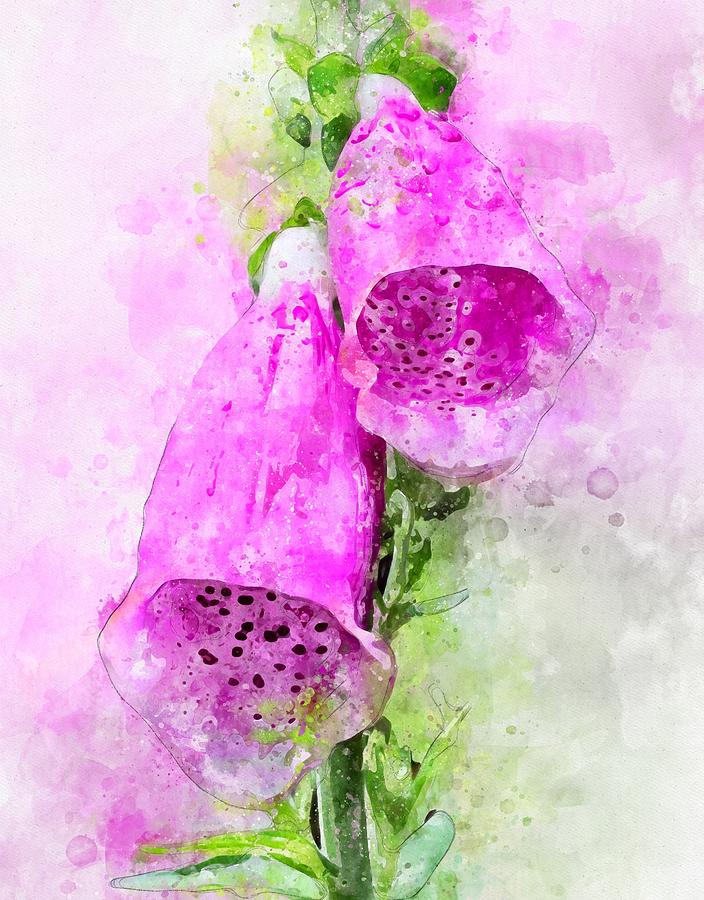The image is a tall, vertically aligned watercolor painting with no border or text. The background is a blend of light purple and white shades at the top and left, fading into light gray and white on the lower right side. Centrally, from the bottom, a green flower stem rises, adorned with several dark green and lighter green leaves. At the top of the stem, two large, bell-shaped flowers droop down on either side. These flowers are primarily bright pink or fuchsia with dark purple specks or black dots inside, presenting a tulip-like shape. The exteriors of the petals blend various hues of pink, purple, and some shades of orange and red, adding depth and vibrancy. The painting employs light ink to outline certain details, enhancing the composition's delicate watercolor effect.